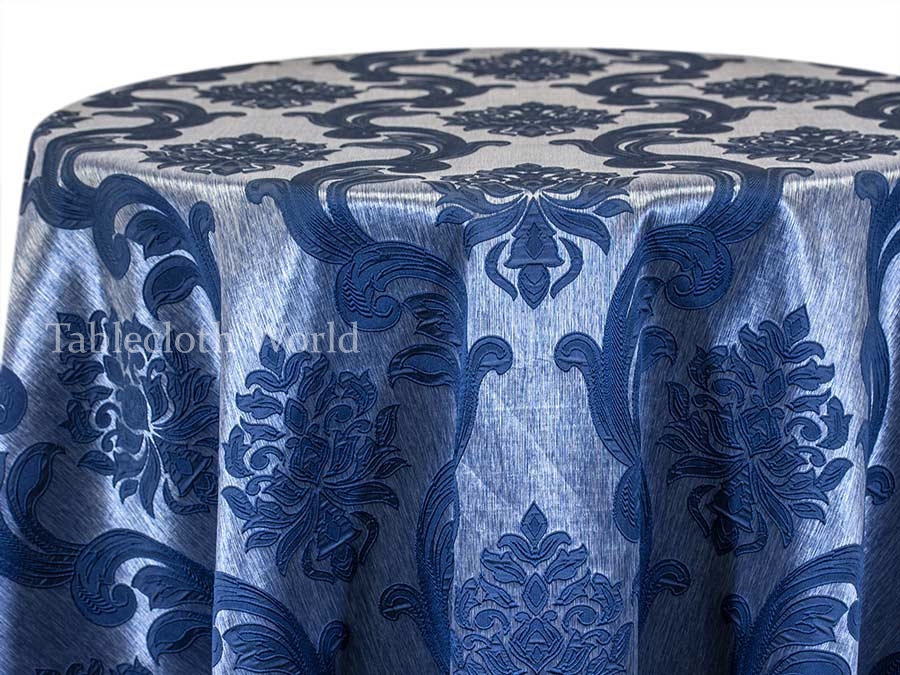The image features a luxurious blue and silver tablecloth draped over a small, round table. The material exudes an air of royalty and nostalgic Victorian elegance, characterized by detailed, ornate floral designs and elegant embroidered patterns that resemble fleur-de-lis symbols. These intricate designs appear to be appliqued onto a lighter blue, textured fabric, with visible vertical fiber stripes contributing to the tablecloth's opulent and eloquent appearance. The top of the table is flat with no items placed on it. You can also notice creases and wrinkles in the tablecloth, adding a touch of realism to the photograph. Positioned toward the middle left side of the image is a watermark that reads "Tablecloth World," identifying the source of the image. The photograph is carefully cropped to focus on the luxurious table setting against a plain white background.